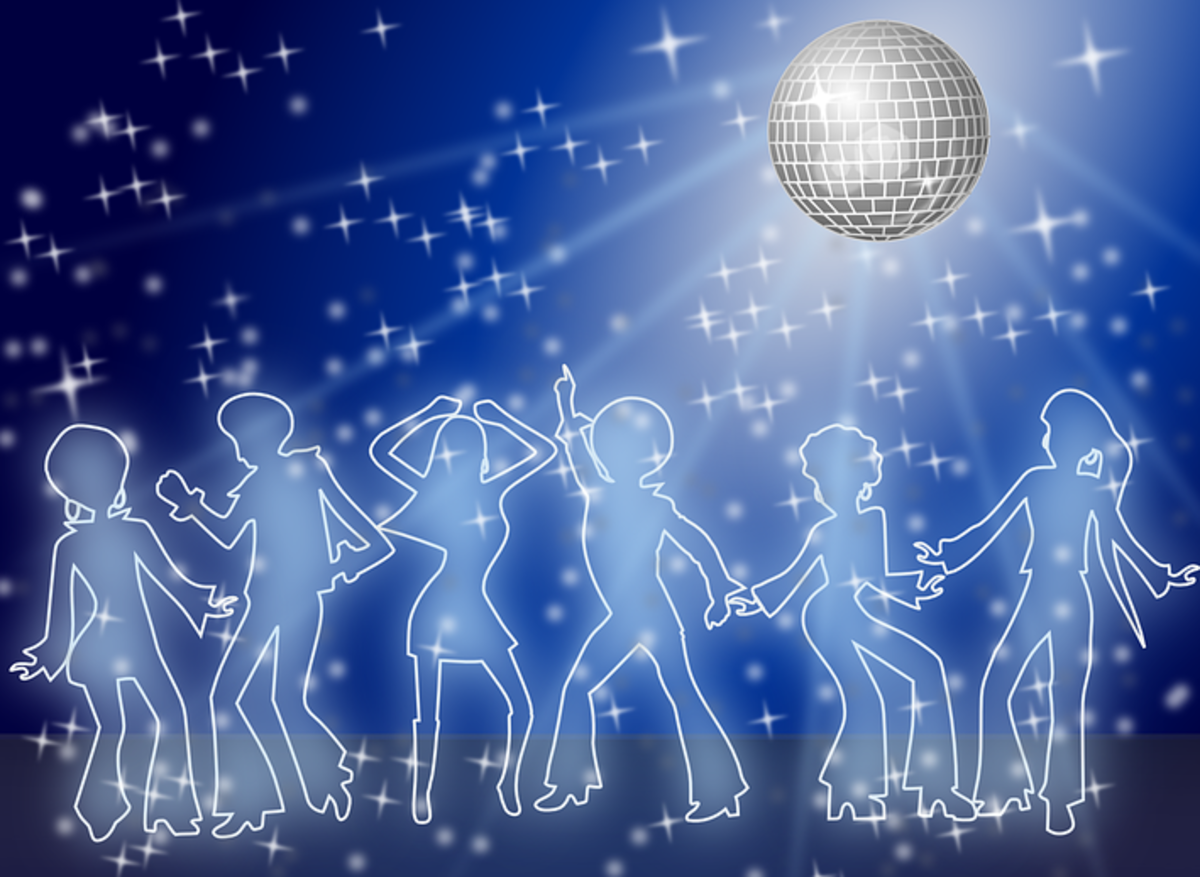The rectangular graphic depicts a vibrant disco scene reminiscent of the 1970s. The background transitions from light blue in the center to deep navy blue at the edges, interspersed with small white, cross-shaped stars that evoke a starry night. Dominating the top right corner is a mirrored disco ball, intricately designed with silver squares and emitting beams of light that radiate in a light blue hue, casting reflective points across the scene.

At the bottom, six featureless figures—drawn as white outlines with light blue interiors—groove to the disco vibe. Their confident poses, including one with hands in the air and another striking a classic disco point, suggest animated dancing. They are wearing high platform shoes, further emphasizing the nostalgic era. The makeshift dance floor beneath them is rendered in gray, providing a subtle base for the silhouetted dancers. The overall composition, devoid of text, artistically captures the energy and ambiance of a lively disco night.